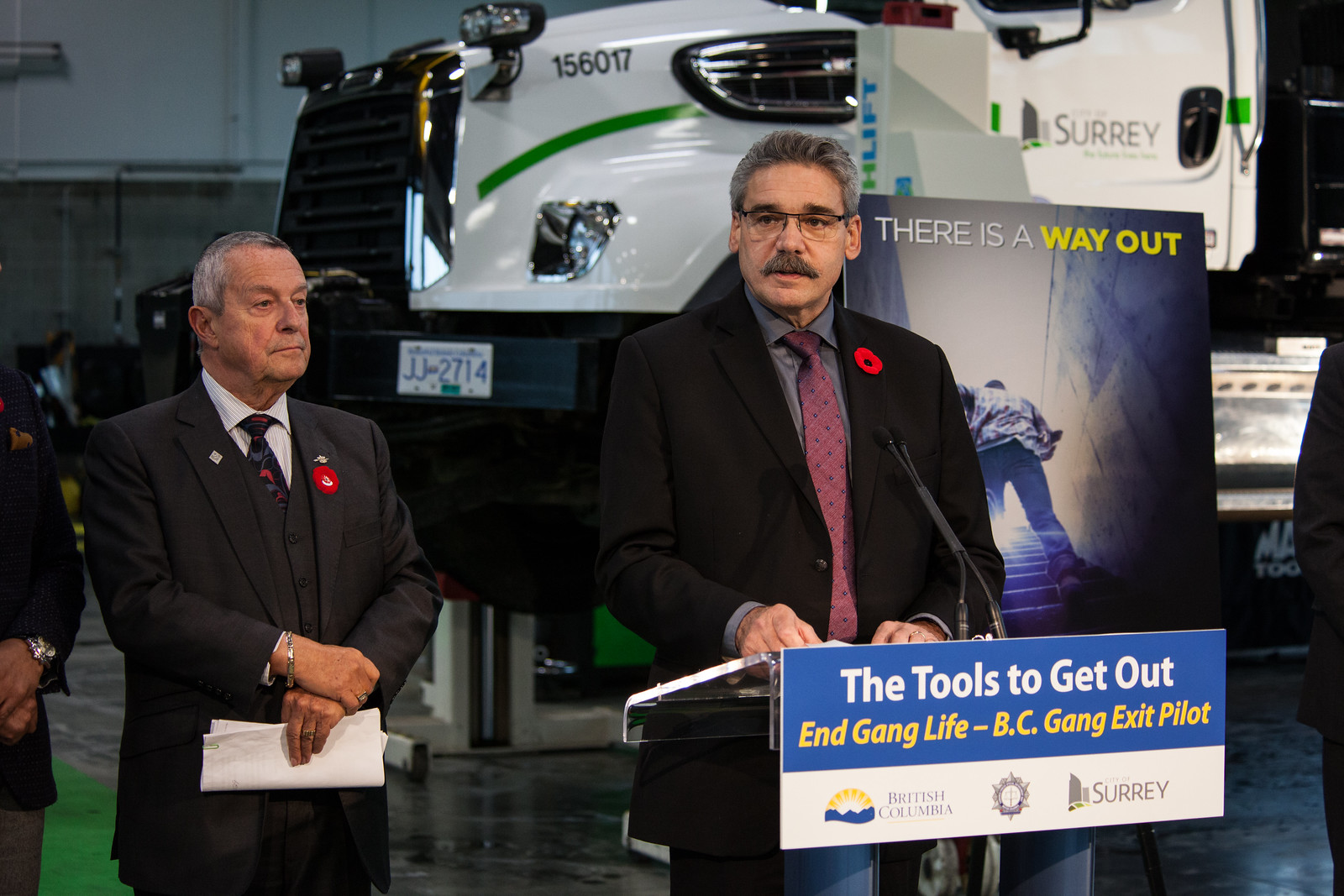The image captures an indoor event, likely a seminar aimed at providing resources for individuals seeking to exit gang life. The setting appears to be within a truck facility. Centered in the image is a man donning a black suit with a white undershirt and a pink tie, speaking at an upright podium equipped with microphones. The podium is adorned with a blue and white sign that reads, "The Tools to Get Out and Gain Life BC, Gang Exit Pilot," along with logos representing British Columbia and local law enforcement. To his left, another man, also in a black suit but with a gray undershirt and a black-and-red tie, stands holding a piece of paper. Both men have gray hair. Behind the speaker, the upper half of the background features the front part of a large truck, and above his left shoulder, there's a poster that conveys the message "There is a way out," illustrated with an image of a man climbing stairs toward a bright light. The setting is completed by a gray-and-white back wall and a floor with green and gray tones. Visible in the background is a license plate labeled JJ2714, enhancing the sense of realism in the scene.